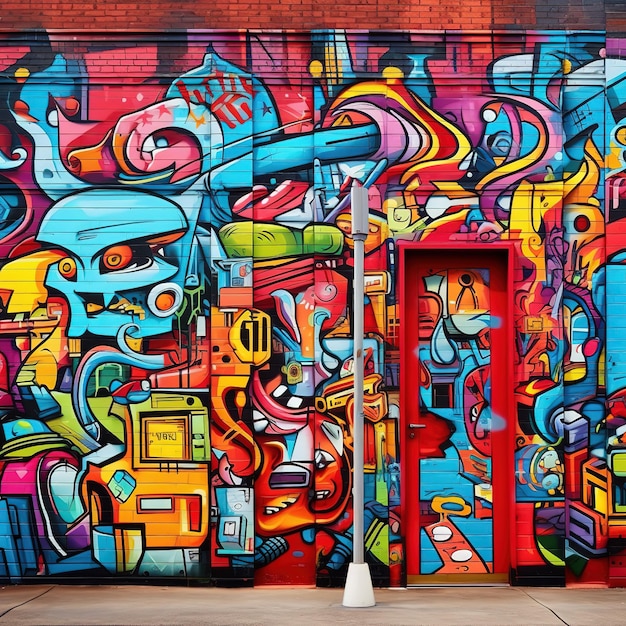This image captures an outdoor scene featuring a brick building adorned with a vibrant mural. The upper portion of the wall displays classic red bricks, while the side boasts an elaborate mural bursting with a spectrum of colors including blue, pink, yellow, orange, dark blue, purple, and green. On the right side of the building, there is a tall, rectangular door fitted with a dark-colored lever handle and framed in red. In the foreground, a street light on a long gray pole stands in front of the building, casting an urban charm. The scene is completed by a gray sidewalk at the base, grounding the dynamic composition.